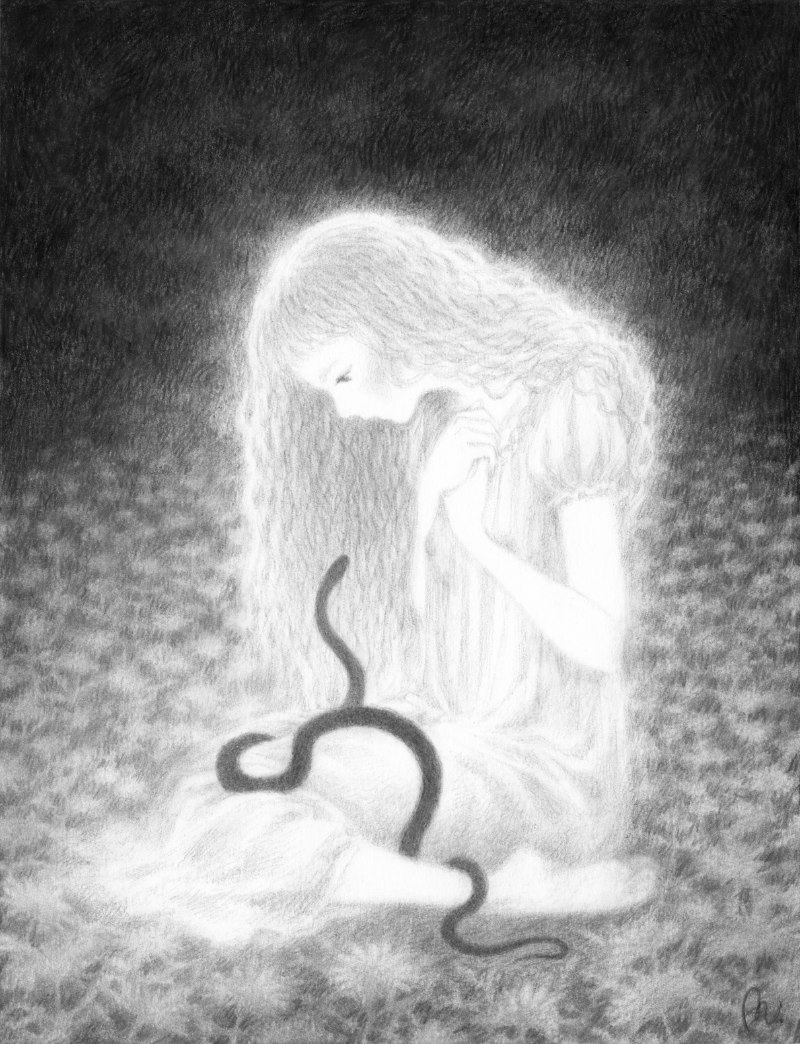This vertical rectangular, monochromatic black-and-white graphic is a striking drawing of a young girl with exceptionally long, dark, curly hair cascading down to her feet. She is sitting barefoot on her knees amidst a field of white daisies, with intricately detailed black eyes and her hands crossed over her chest. Her glowing, luminous form has a slightly transparent quality, particularly in her hair. She is dressed in a long, short-sleeved nightgown that drapes past her knees.

Entwined with the girl is a sinister black two-headed snake. One head is coiled around her leg and is starting to ascend toward her face, while the other head curves mysteriously behind her, its destination unseen. The background of the image is mostly dark with subtle gray shapes, creating a stark contrast that enhances the ethereal quality of the young girl. Though a name appears at the bottom of the picture, it is indecipherable. The overall scene is hauntingly beautiful, with the interplay of light and dark elements drawing the viewer’s eye to the central, almost holographic, figure of the girl and her serpentine companion.